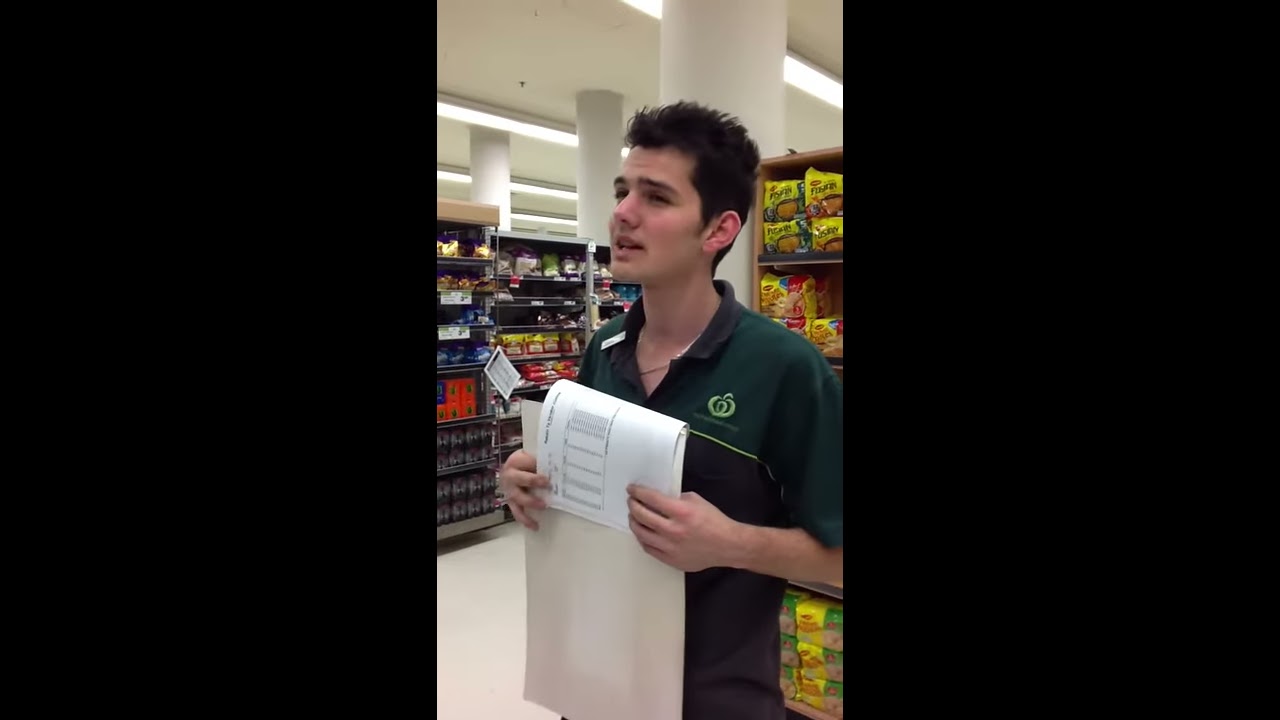In the image, we see a man inside a grocery store, holding a paper up to his chest. He has spiky black hair, approximately three inches long, and light skin. His mouth is open, revealing the tips of his top and bottom teeth as he speaks, with his eyes slightly squinted, suggesting he's engaged in a conversation. The man is wearing a green collared shirt that features a black-colored collar. On the left side of his chest from our viewpoint, there's a name tag. On the right side, there's a lighter green apple symbol. 

The paper he is holding appears to be a spreadsheet with five main columns, and it's folded at the top where his hands grip it. He uses both hands to hold the paper, which faces mostly toward him. Behind the man, there are shelves stocked with various food items, including what seem to be crackers or snacks. In the left background, another grocery aisle with more food items is visible. Additionally, the store features tall white pillars that extend from the floor to the ceiling, with all-white ceilings giving the space a clean and organized look. The overall setting suggests that the man might be taking inventory or managing stock.